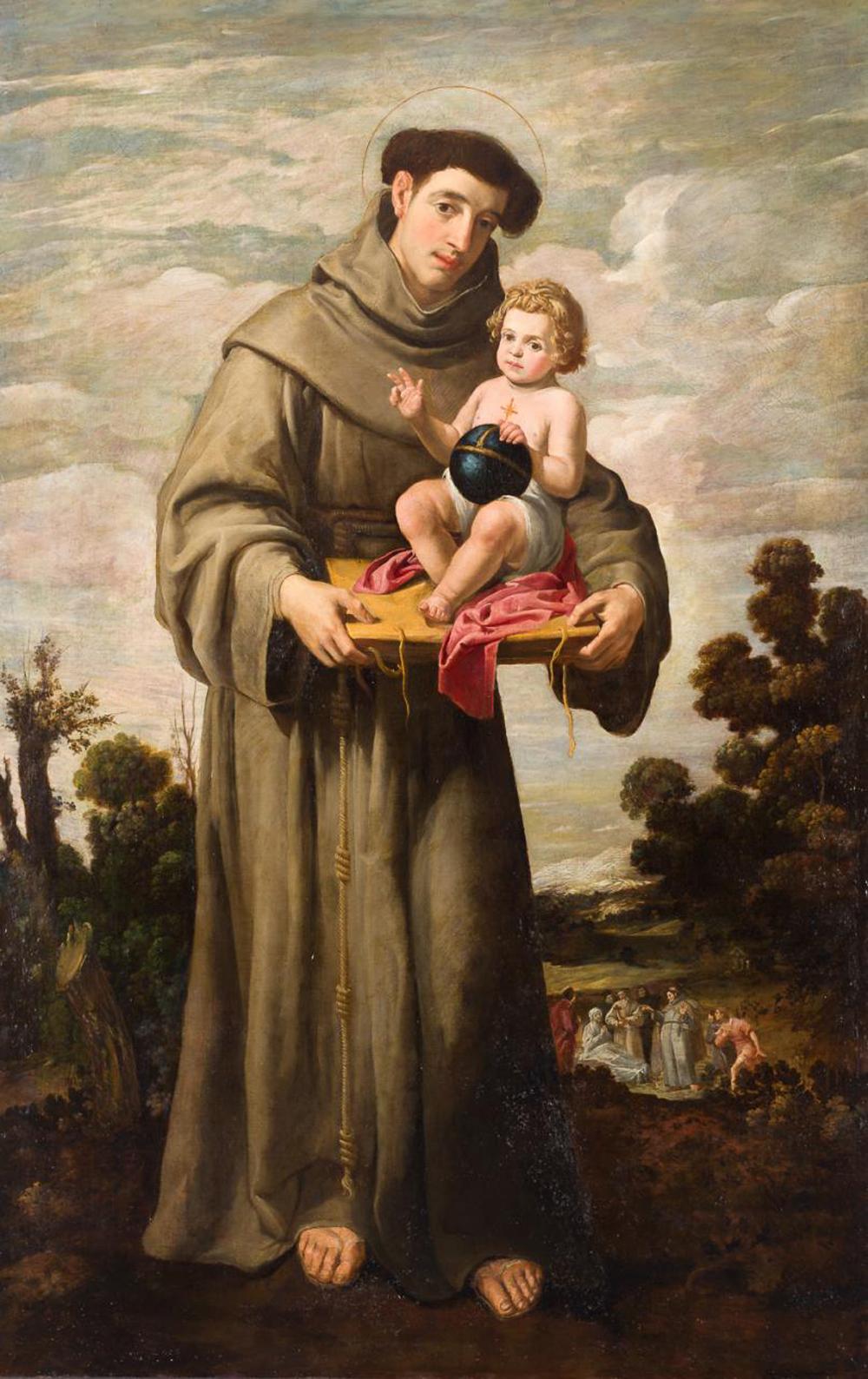This is a detailed description of a vertically aligned rectangular painting depicting a religious scene. At its center is a holy man, likely a monk or a holy figure, with brown, somewhat long hair. He wears grayish-brown monk robes that reach the ground and has bare feet. This man is holding a rectangular brown object, possibly a platform or a book, upon which a baby is seated. The baby, thought to represent Christ, has curly golden locks and is lightly clothed in a white diaper with a cross necklace around its neck, signifying a christening or baptism. The baby is also holding a black orb with a cross on top and has one hand raised with two fingers extended in a gesture of blessing.

In the background, lush vegetation, including green trees, can be seen on both sides. The upper half of the artwork features a vast sky filled with fluffy clouds in shades of white, gray, and brown. The bottom right corner depicts a group of figures dressed in robes, perhaps elegant women or other holy individuals, who are gathered at a distance, adding depth to the scene. The painting’s color palette includes black, white, gray, brown, pink, red, gold, yellow, green, olive, and tan, enhancing the detailed and serene composition of this religious artwork.